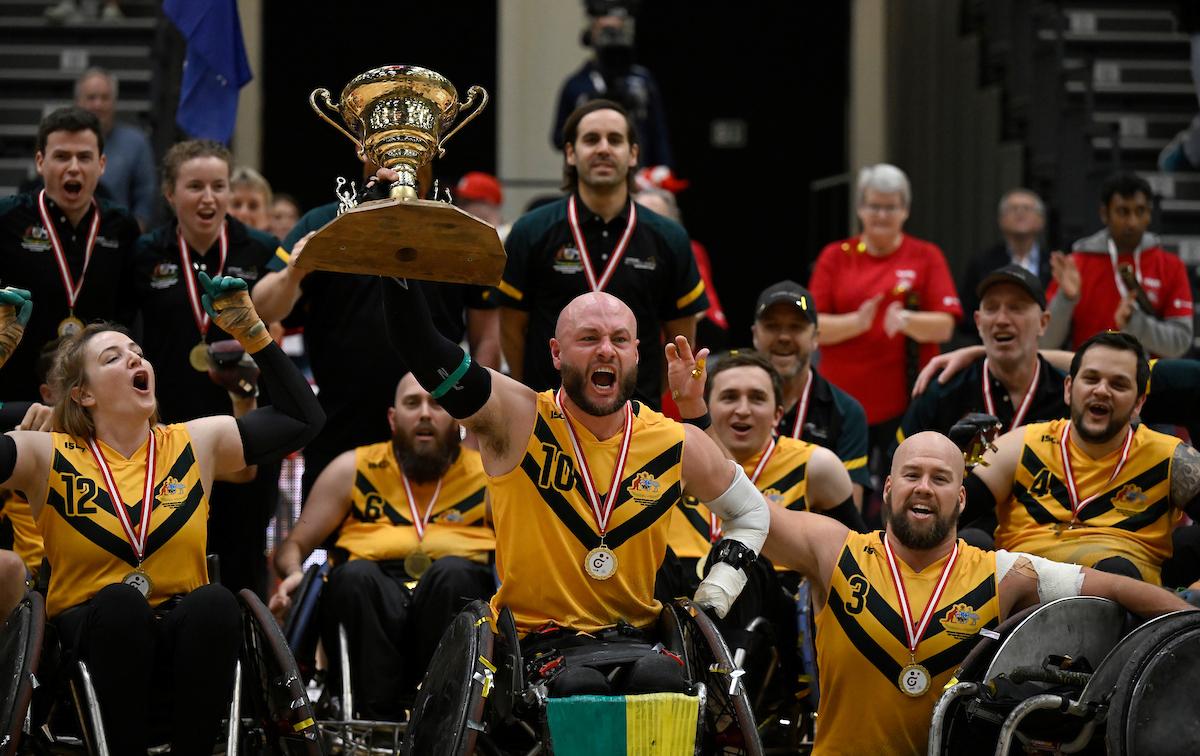The image depicts a jubilant wheelchair basketball team celebrating their victory in an indoor auditorium. All team members are seated in their wheelchairs and donning gold and black uniforms with red and white lanyards carrying medals around their necks. At the center of the team is a bald man with a thick beard, proudly hoisting a large, golden cup trophy aloft. He is surrounded by five other teammates, a mix of men and women, all rejoicing with raised hands and beads of excitement. Behind them, coaches in black button-up jerseys and baseball caps, also adorned with medals, share in the celebration. The background displays clapping spectators and a clear sight of bleachers, indicating a post-game victory. The photograph captures the elation of the team and their supporters, though the team's name and nationality remain unidentified.